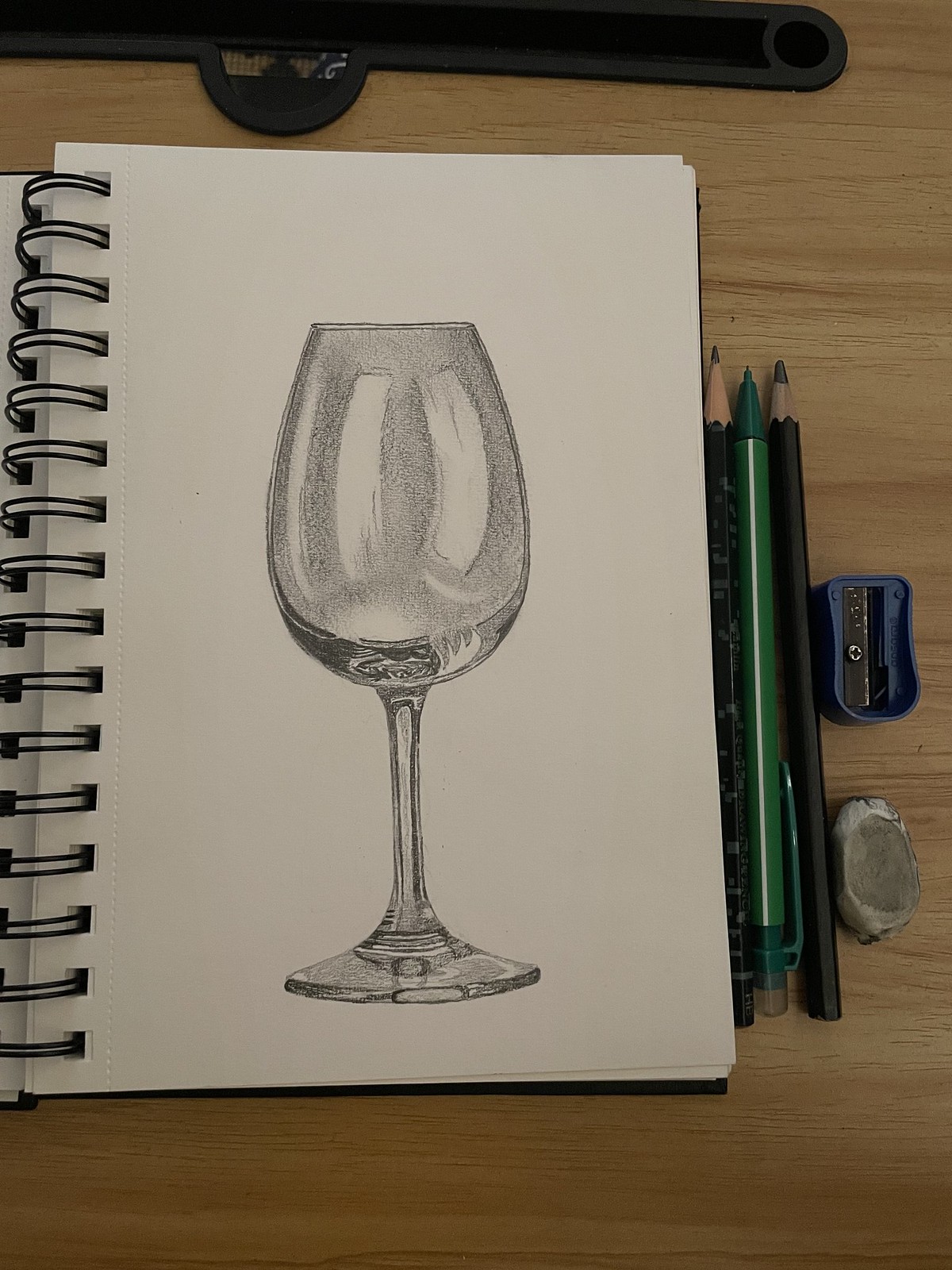The image depicts a neatly arranged drawing workspace on a desk. At the center of the desk lies a drawing book with a ring binding on the left side, clearly indicating that it is a sketchbook. The sketchbook is open to a page featuring a detailed black-and-white pencil drawing of a wine glass. The wine glass illustration is meticulously done, with careful shading that highlights its reflective surfaces, particularly emphasizing the vertical gleams that suggest the glass is catching light. Furthermore, there are smaller shine spots illustrated on the stem and base of the glass, adding to the realism of the drawing.

To the right of the drawing book, a variety of drawing tools are laid out in an orderly manner. There are three colored pencils, each in a different hue, alongside three standard graphite pencils. Additionally, there is a pen equipped with an eraser, as well as a small pencil sharpener, indicating readiness for continued artistic work. The overall scene conveys a sense of calm focus, ideal for creativity and precision in drawing.